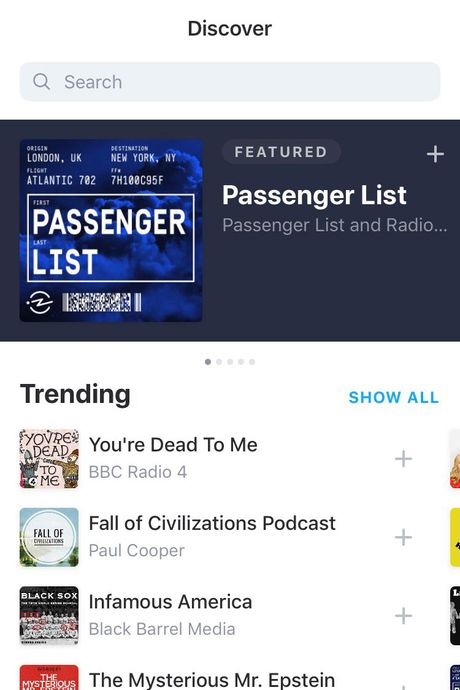The interface displays a variety of elements designed to help users discover and search for content. At the top center, there's a "Discover" section. Directly below it, a gray search bar reads "searching gray" and includes a search icon. Underneath the search bar, the section titled "Featured" appears, introducing highlighted content like "Passenger Lists" and "Passenger List and Radio." There's a plus icon located in the upper right corner.

Beneath this, there are navigation dots, suggesting additional images are available if you swipe right. The current view indicates you're on the first dot out of five. The left side says "Trending," and on the right, "Show All" is highlighted in a turquoise color. 

Four images are displayed in a row below this section, with the bottom images partially cut off. To the right of the top-left image, there is a title and description: "You're Dead to Me" from BBC Radio 4, accompanied by a gray plus sign. Next to the second image, it reads "Fall of Civilizations Podcast" by Paul Cooper, also with a plus sign. The third image lists "Infamous America" by Black Barrel Media, again with a plus sign. The fourth image, which is cut off, titled "The Mysterious Mr. Epstein."

The color scheme includes various shades of black, gray, white, blue, pink, red, yellow, and turquoise, creating a visually engaging interface.